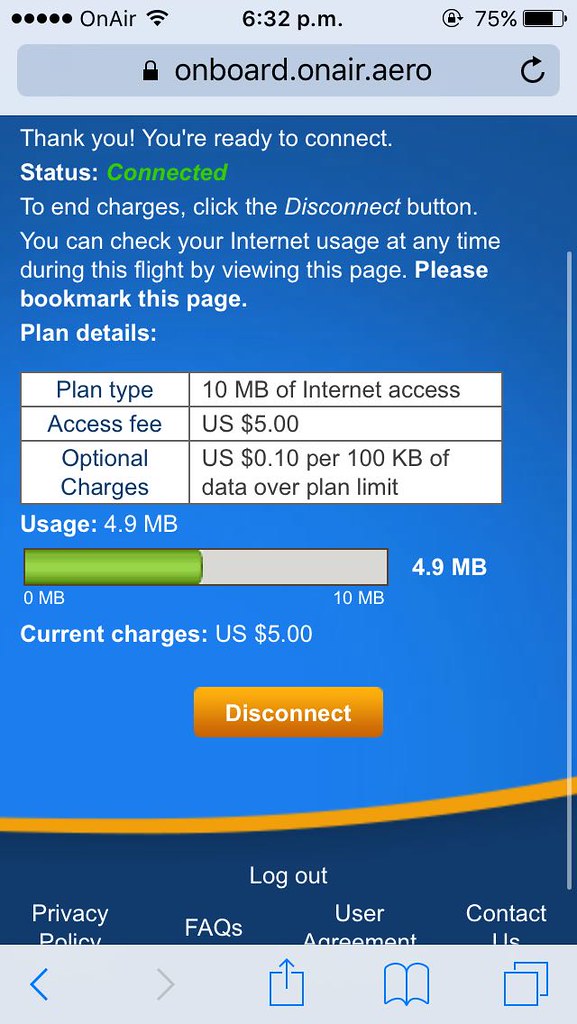The image is a detailed screenshot taken from a mobile phone, displaying an in-flight internet connection status and details. The display is predominantly vertical. At the top, there is a light blue border with a dark blue search bar in the center, featuring a black lock icon and the URL "onboard.onair.aero" with a refresh symbol. Above the search bar, from left to right, are five solid black dots followed by the text "On Air," the time "6:32 p.m." in the center, and a battery icon showing 75% charge. 

Beneath this header, the main screen is primarily blue, displaying connection information in white text. It reads: "Thank you. You're ready to connect. Status: Connected" with "Connected" highlighted in green. The text continues, "To end charges, click the disconnect button. You can check your internet usage at any time during this flight by viewing this page. Please bookmark this page." Under "Plan details," it specifies the plan type: "10 MB of internet access," the access fee: "U.S. $5," and optional charges: "U.S. $0.10 per 100 KB of data over the plan limit." 

A white rectangular section shows the plan usage: "4.5 MB out of 10 MB" and the current charge: "U.S. $5." At the bottom, there's an orange rectangle with "Disconnect" in white text. Below, a blue border with various options in white text reads: "Log out, Privacy Policies, FAQs, User Agreement, Contact Us." The very bottom features a light blue or gray border with navigation buttons: back, forward, upload, bookmark, and open pages.